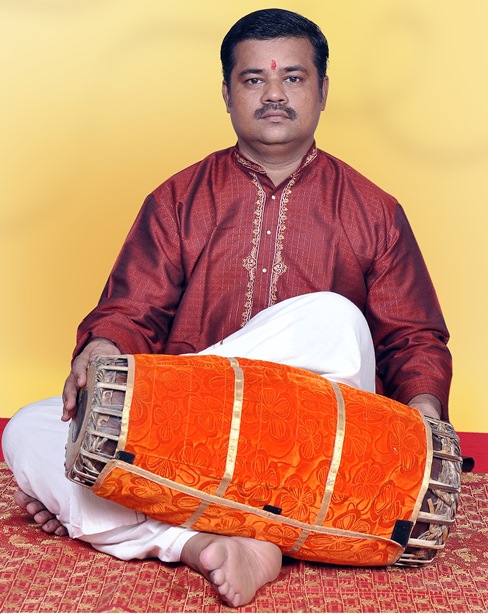The photograph captures an Indian man seated barefoot in a meditative pose on a red and gold patterned carpet. The man has short black hair and a thin mustache, accentuated by a red dot on his forehead between his dark eyebrows. His attire consists of white pants and a burnt orange traditional long-sleeve button-down shirt adorned with gold trim around the chest area. Leaning on his bare foot is a traditional drum, resembling a wooden barrel wrapped in orange patterned fabric, lying horizontally. A solid yellow wall serves as a vibrant backdrop. His gaze is fixed directly at the camera, maintaining a serious expression.